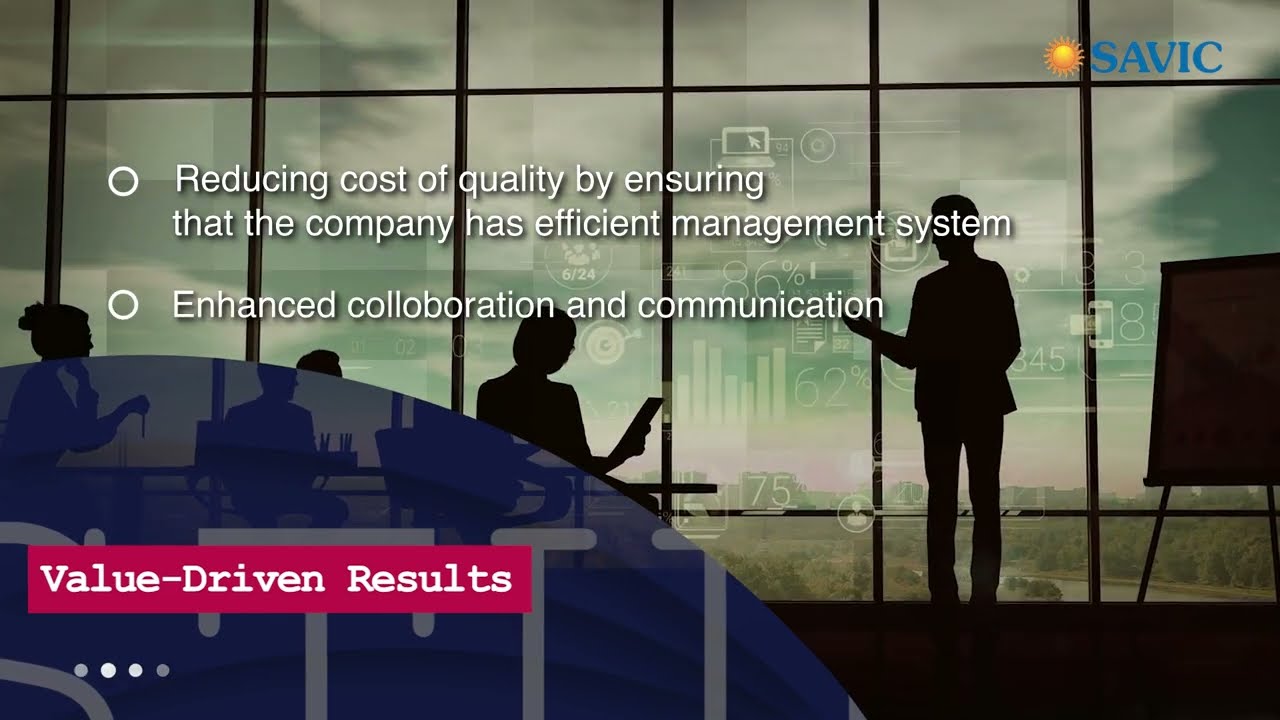The image is a PowerPoint slide from a presentation, featuring two main bullet points. The background displays silhouettes of people in a board meeting, with a person standing on the right next to a bullet-point chart. The chart has two key points in white text: "Reducing cost of quality by ensuring that the company has efficient management system" and "Enhanced collaboration and communication," albeit with a spelling error in "collaboration" (spelled "l-c-o-l-l-o-b-o-r-a-t-i-o-n"). In the lower left corner, there's a red rectangle containing the phrase "Value-driven results" in white typewriter-style font. A blue semicircle shape is partially visible behind this red rectangle. Additionally, in the top right corner, there is a logo of an orange sun with the word "SAVIC" in blue letters. The overall scene suggests a corporate setting aimed at highlighting the company's strengths in management efficiency and collaboration to deliver value-driven results.